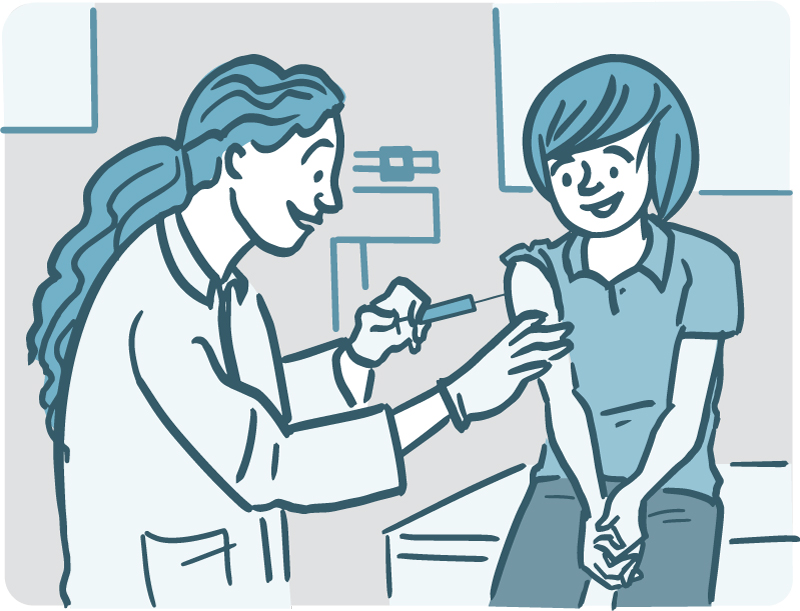In this detailed cartoon illustration, set in a doctor's office, a female doctor with long blue hair pulled back into a ponytail is administering an injection into the right arm of a young woman who is sitting on an examination table. The doctor is wearing a white coat and is holding the needle in her left hand while steadying the patient’s arm with her right hand. The young woman, who is dressed in a blue shirt with the sleeve rolled up to her shoulder, has her hands clasped in front of her and is looking down at the injection with a smile. Both the doctor and the patient are smiling, conveying a calm and reassuring atmosphere. In the background, there is a weight scale and two white squares with blue outlines on the wall, adding to the clinical setting. The entire scene is illustrated in shades of blue and white, enhancing the medical theme of the image.